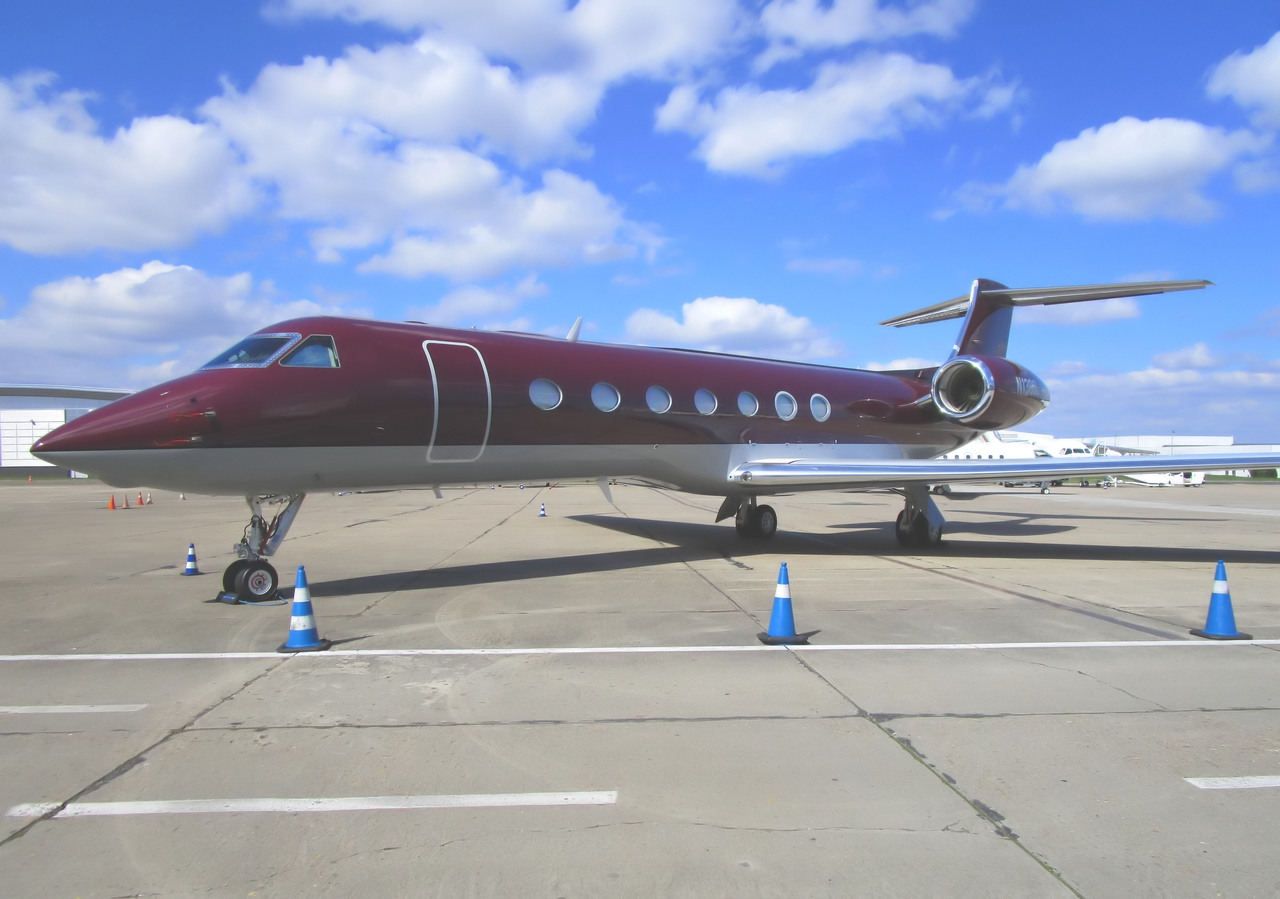This photograph captures a meticulously detailed scene of a burgundy-colored Learjet parked on the gray tarmac of an airport. The jet's sleek body features a two-tone design, with the top two-thirds painted in a striking maroon hue and the bottom third in a gleaming silver. The aircraft has seven porthole-style passenger windows, with an equal number likely on the opposite side. It stands upright on its three-part landing gear, which includes a wheel under each wing and one at the front. The jet's engines are mounted at the rear of the body, contributing to its streamlined appearance, while the tail section includes a vertical fin and two horizontal stabilizers extending sideways.

In the foreground, three blue safety cones are lined up in front of the jet, adding a splash of color to the asphalt surface. The expansive tarmac, painted in parts, stretches out under a clear, azure sky dotted with scattered clouds. Additional white aircraft are visible in the background, hinting at a bustling airport environment. The setting appears to be a private section of the airport, likely intended for private jets, given the presence of multiple aircraft and the orderly layout. Overall, this image encapsulates the elegance and sophistication of a private jet on a bright, sunny day, with an immaculate blue sky overhead and other elements complementing the primary focus of the Learjet.